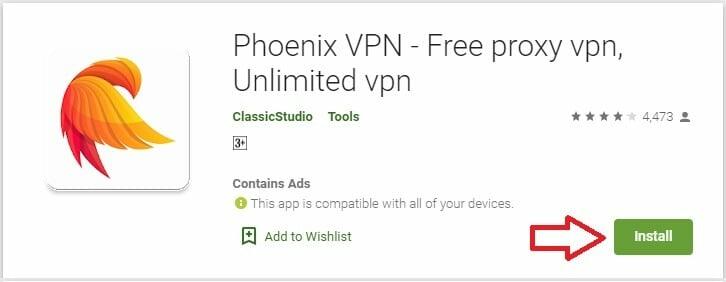The image appears to be a screenshot taken from either the Google Play Store or a similar website, displaying the details of an app. The background is completely white.

In the top left corner, there is a white box with a thin gray outline, featuring a close-up side view of a stylized bird. The bird resembles a mythical phoenix, with an orange wing, a red tail, and a partially visible face and beak, depicted in a silhouette. 

Above the bird, in thin black font, the app name "Phoenix VPN-FreeProxy" is displayed in capital letters, followed by "VPN, unlimited VPN" in lowercase. Beneath this text, "ClassicStudio" is written in small green font, followed by the word "Tools." The app is rated four out of five stars based on 4,473 reviews, as indicated by a star rating system.

Adjacent to "ClassicStudio," a note specifies that the app "contains ads," marked by a small green circle with a white exclamation mark inside.

There is a statement in gray text informing that the app is compatible with all of the user's devices. Next to this, a bookmark icon and the phrase "add to wishlist" are present. 

Toward the bottom right, a large, hollow red arrow points towards a green box containing the word "Install" in white letters, indicating the button to download the app.